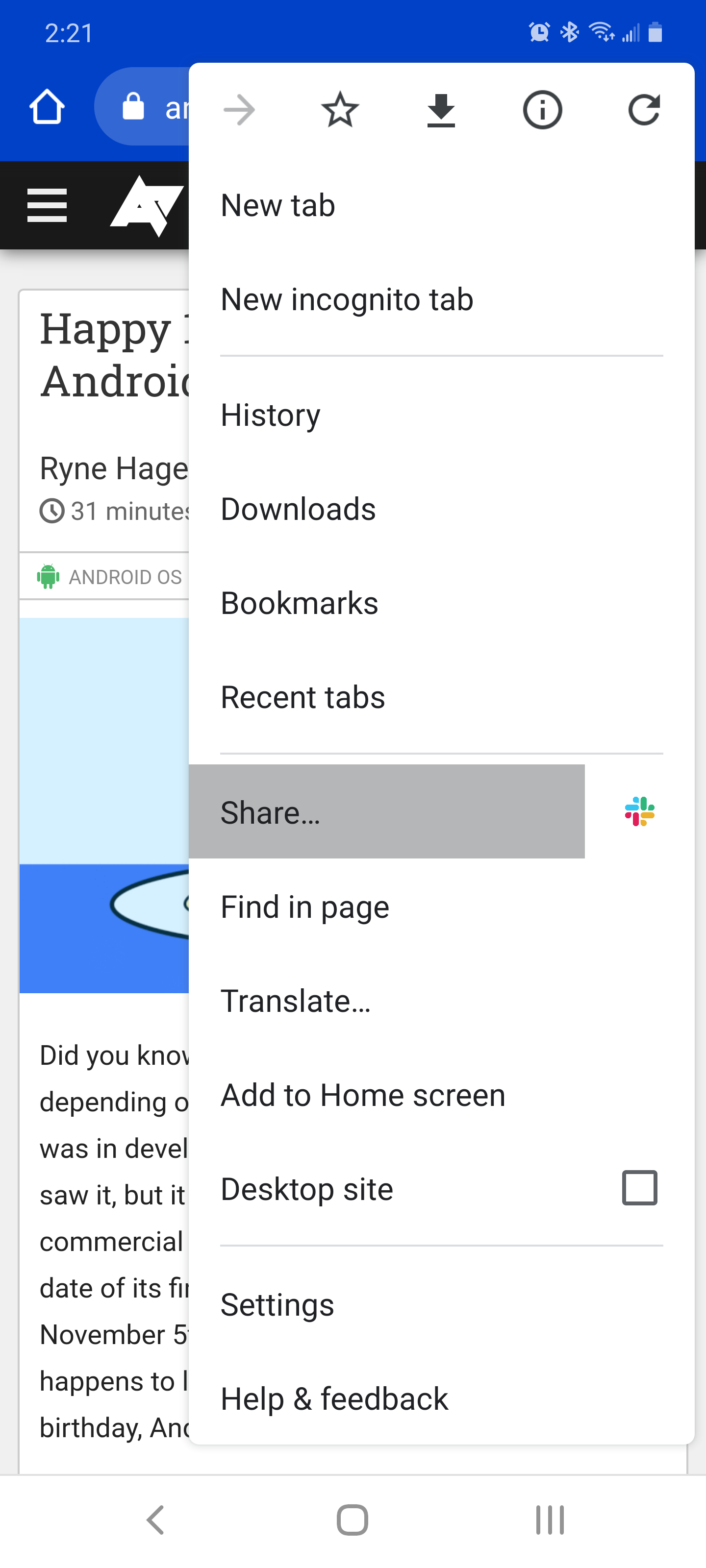In this detailed image caption, we explore a mixture of digital interface elements and personal context:

The image illustrates a multitude of visual elements commonly found within a smartphone's operating system interface, specifically targeting Android OS. The interface includes a visible battery icon, indicating the device's power status, alongside a Bluetooth symbol and Wi-Fi signal strength indicator, showcasing the connectivity options available. Additionally, there is a home padlock icon, signaling device security, and a star icon typically used for bookmarking favorite items.

A prominent download button is highlighted, indicating ongoing or recent downloads which seem to include a history, bookmarks, and recent tabs options. Three horizontal lines, known as the “hamburger menu,” appear in the image, suggesting additional menu options available for exploration. This menu might allow the user to open a new tab, initiate a new incognito browsing session, view browsing history, share content, and perform other actions such as finding a specific term on a page, translating text, or adding a webpage to the home screen.

The image also features two blue squares with an embedded oval piece, possibly representing an app or folder. Other notable icons include an arrow for navigation purposes, a refresh symbol to reload content, and a flower icon colored in blue, red, green, and yellow - likely representing a multitasking or sharing functionality.

The illustration marks a "share" feature highlighted in gray, indicative of a currently selected or active mode. Mention of a person named Ryan Hage, with a timestamp of 31 minutes and association with an Android device, suggests interaction with the mobile content or an action taken.

Furthermore, there are references to system settings including options like 'Find in Page,' 'Translate,' 'Add to Home Screen,' and 'Desktop Site,' each designed to enhance user interaction within the mobile browser.

There is a mention of November 5 as a date of significance, possibly a birthday, coupled with an assistance and feedback section indicated by the "help and feedback" terms, providing users support and troubleshooting options.

Overall, this detailed caption thoroughly captures the myriad of Android operating system features seen within the mobile interface, interspersed with personal elements and context.